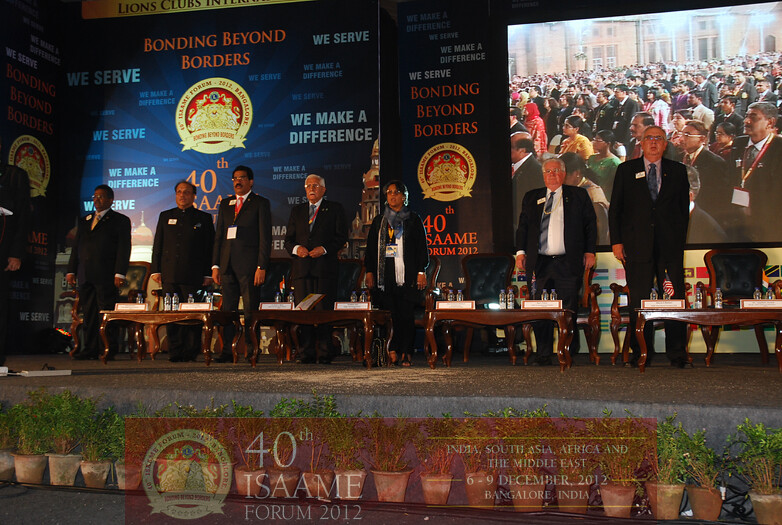In this photograph, a group of approximately eight or nine people, predominantly men, are standing on a stage arranged in a line. Each person is dressed formally in suits with varying colors of ties, including yellow, red, blue, and gray. The woman in the group is wearing a blue or gray scarf along with a yellow badge around her neck. A notable feature is an individual in a black suit adorned with a gold chain draped from lapel to lapel.

In front of the group, three low wooden tables serve as a podium, with objects such as bottles of water, little flags, and white boxes placed upon them. The tables have brown chairs with blue backings positioned behind them. The stage, which is about three to four feet off the ground, is adorned at its base with twenty flower pots containing lush green ferns, adding a touch of nature to the setting.

Behind the group, a large backdrop features several inscriptions. Prominently displayed in orange is the phrase "Bonding Beyond Borders," followed by "We Serve, We Make a Difference" written in blue. There is also a mention of the "40th Anniversary," with detailed text specifying "India, South Asia, Africa, and the Middle East, 6 to 9 December 2012, Bangalore, India." The backdrop includes a seal with gold, red, and some symbolic imagery, and the words "Lions Club" in black on a gold background at the top.

This image appears to capture a ceremonial event, likely an award ceremony or a significant anniversary celebration held by the Lions Club, marked by its international participants and formal setting.